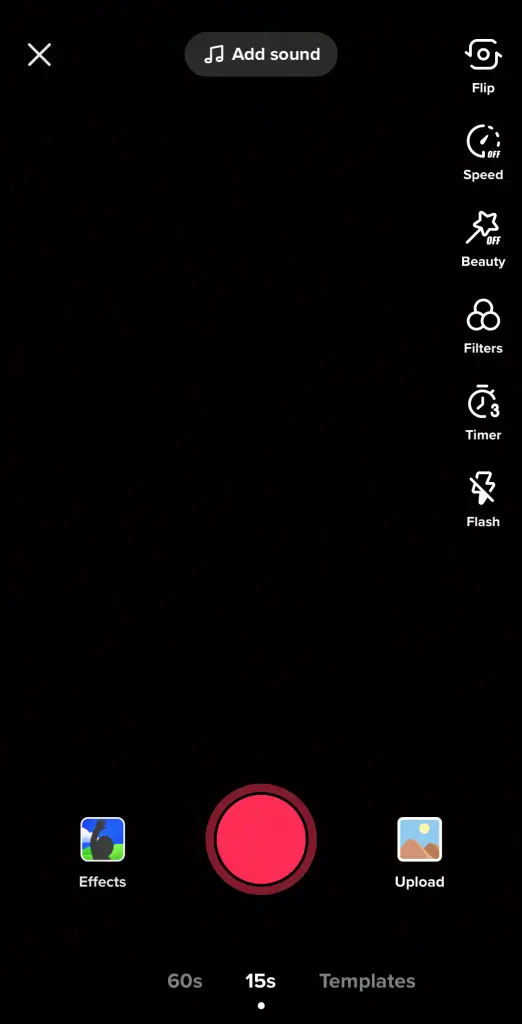The image depicts the interface of a video recording application on a solid black background. In the upper left corner, there is a white 'X'. To its right, there's a gray oval bar with a white music icon and the text "Add Sound" inside it. Further to the right, aligned horizontally, there are six white-labeled options: "Flip," "Speed," "Beauty," "Filters," "Timer," and "Flash," each accompanied by distinct icons. 

- The "Flip" option features an icon resembling an Instagram interface with dashes.
- "Speed" is denoted by a speedometer icon and is labeled "Off".
- "Beauty" is represented by a wand icon and also marked "Off".
- "Filters" show a trio of circles.
- "Timer" is indicated by a timer icon beside the number "3".
- "Flash" depicts a lightning bolt with a slash through it.

Below this set, there are three additional options in white font. The first is "Effects," accompanied by a boxed icon of a figure waving against a sky-blue and green background, symbolizing the sky and ground. To its right is "Upload," indicated by an icon of a square box containing two brown mountains and a yellow sun. Central to these options, there is a prominent red circle.

At the bottom, the screen offers the duration choices "60s," "15s," and "Templates," with "15s" being highlighted by a small white dot.